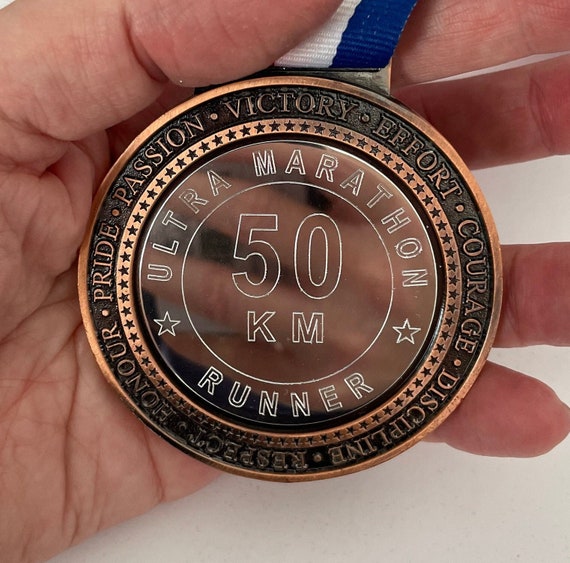A man's hand, with white skin, is shown holding a bronze-colored, semi-translucent medal in a close-up photograph. The medal, which is partially transparent and reflective, captures the faint image of the person’s hand and phone. Encircling its center are the words "Ultra Marathon 50K Runner." Around the edges, inscribed in a clockwise fashion, are the motivational words: Pride, Passion, Victory, Effort, Courage, Discipline, Respect, Honor, separated by stars. The medal is attached to a blue and white striped ribbon, of which only a small section is visible. The background behind the hand is white, highlighting the details of the medal.